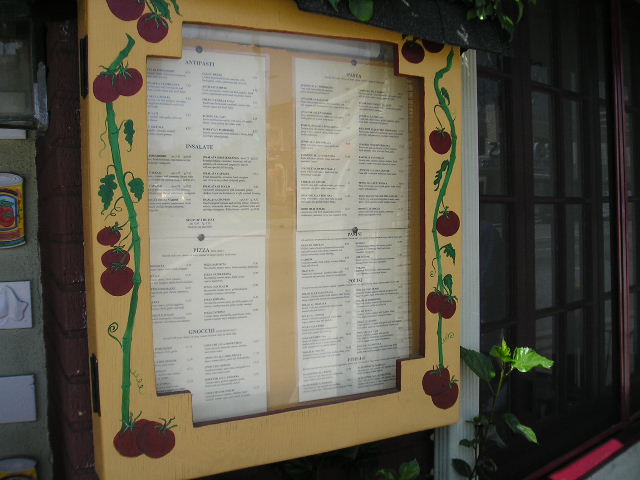This image showcases an outdoor menu board framed with hand-painted cherry tomatoes. The frame features larger black corners and encases a light yellow background. Four sheets of paper, displaying menus with various lines of script, are tacked onto a cork board inside the frame, allowing for easy updates. Positioned next to a dark wooden door with glass panels, the scene is bathed in gentle sunlight that also illuminates a nearby plant. The setting exudes a quaint and inviting atmosphere.